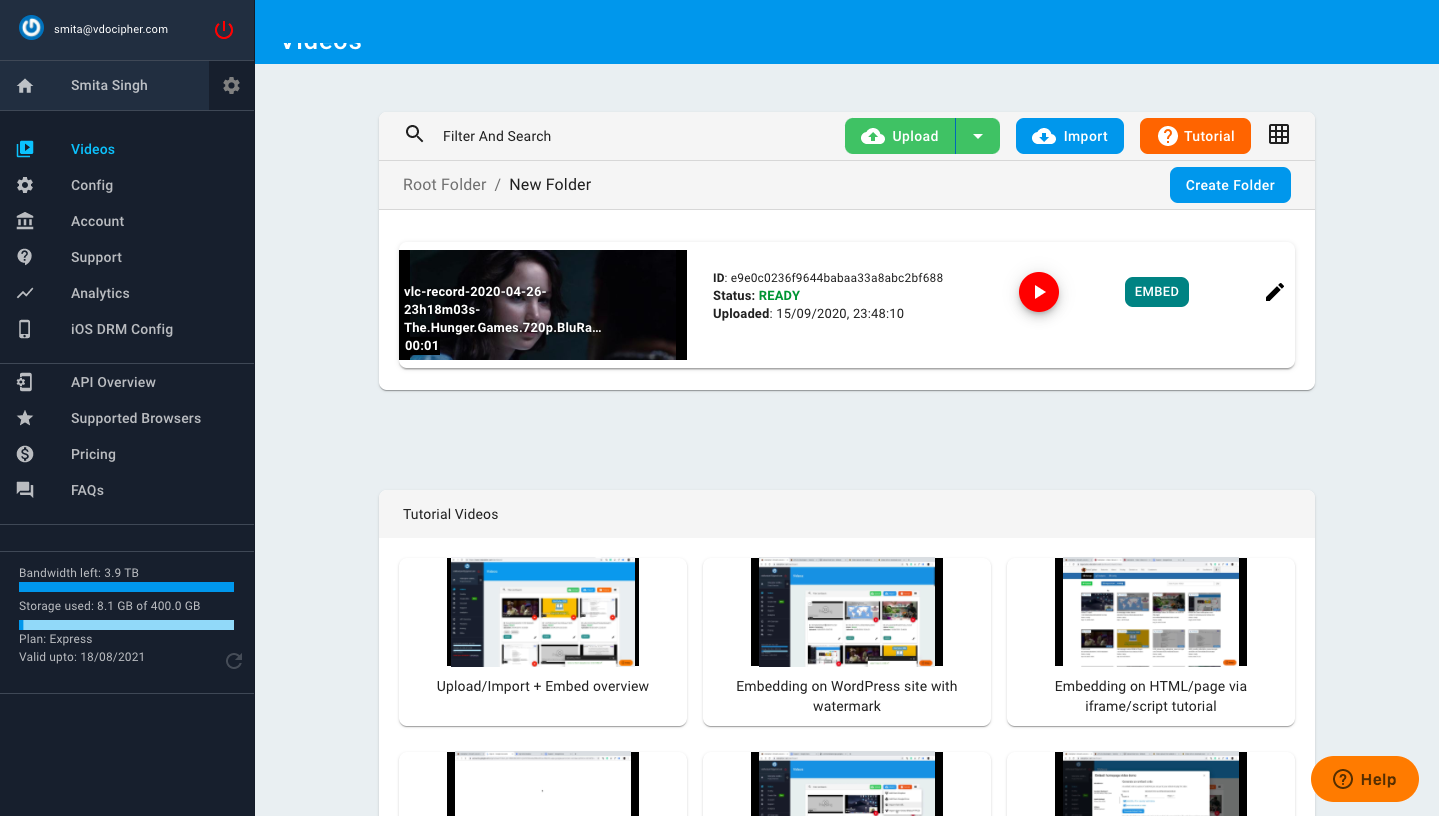In the left section of the image, the background is black. Adjacent to this, there is an image of a house icon next to the name "SMITA SINGH" written in large, block letters. Below this, the word "VIDEOS" appears in blue text. 

Further down, there's an image of a wheel icon, symbolizing settings, followed by menu items labeled "CONFIG," "Account," "Support," "Analytics," "iOS DRM Config," "API Overview," "Supported Browsers," "Pricing," and "FAQ." 

A long blue line stretches horizontally across this section. Above the line, the words "Bandwidth" and "Storage Used" are displayed, with their respective indicators in light blue.

At the center of the image, there is a still from "The Hunger Games" movie, focusing on Jennifer Lawrence's face. Overlaid in white text, it reads "The Hunger Games .720p Blu-ray" and the identifier "001." The status of the file is indicated as "Ready" in green text. Below this information, it states "Uploaded: 15-09-2020," next to an icon of an arrow inside a red circle, which serves as the play button.

Above the movie image, there are three options: "Upload," "Import," and "Tutorial," for user interactions.